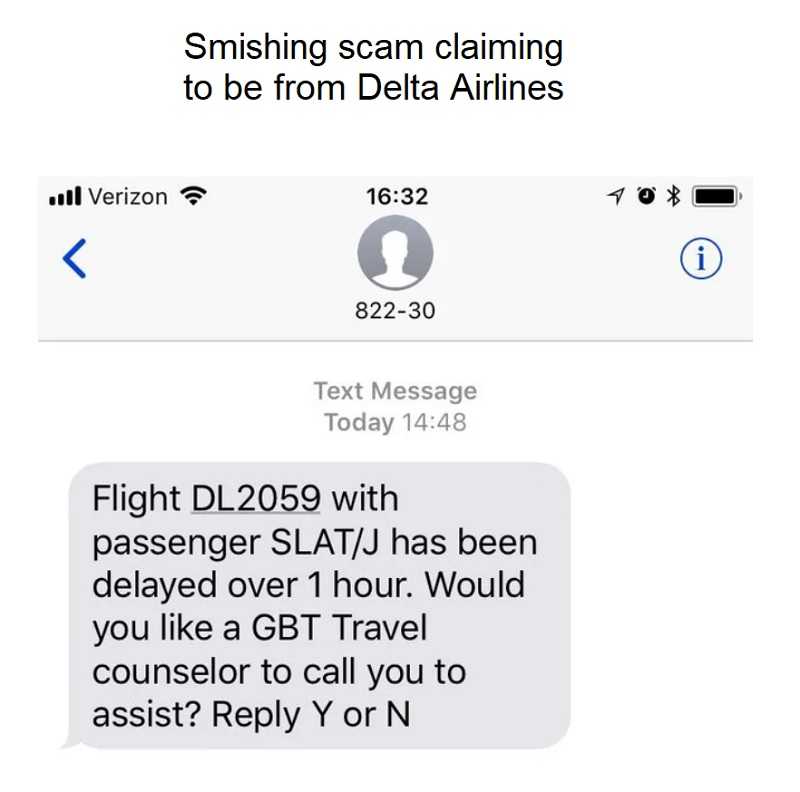**Detailed Caption:**

The image is a screenshot of a smartphone displaying a suspicious text message on a white background. The top part of the image shows the status bar with details indicating a Verizon Wi-Fi connection, a time of 16:32, location services, alarm set, Bluetooth enabled, and a full battery icon. Positioned below the status bar is a blue arrow pointing to the left, and a generic profile picture followed by the identifier "3822-30". On the right side of this section, there is a blue circle with a white eye icon in its center.

The text message appears below this header with a timestamp of 14:48. The content of the message reads: "Flight DL2059 with passengers lat/J has been delayed over one hour. Would you like a GBT travel counselor to call you to assist? Reply Y or N." The message is presented in a standard gray and black text on a white background, with the only additional color being blue used for elements such as the arrow and the eye icon.

This screenshot was likely taken to capture evidence of what appears to be a smishing scam, falsely claiming to be from Delta Airlines. The scammers are attempting to deceive the recipient into replying to the message. The overall color scheme of the image consists primarily of blue, gray, black, and white.

Given the blatant attempt to exploit the recipient, receiving such a message would indeed be frustrating and concerning.